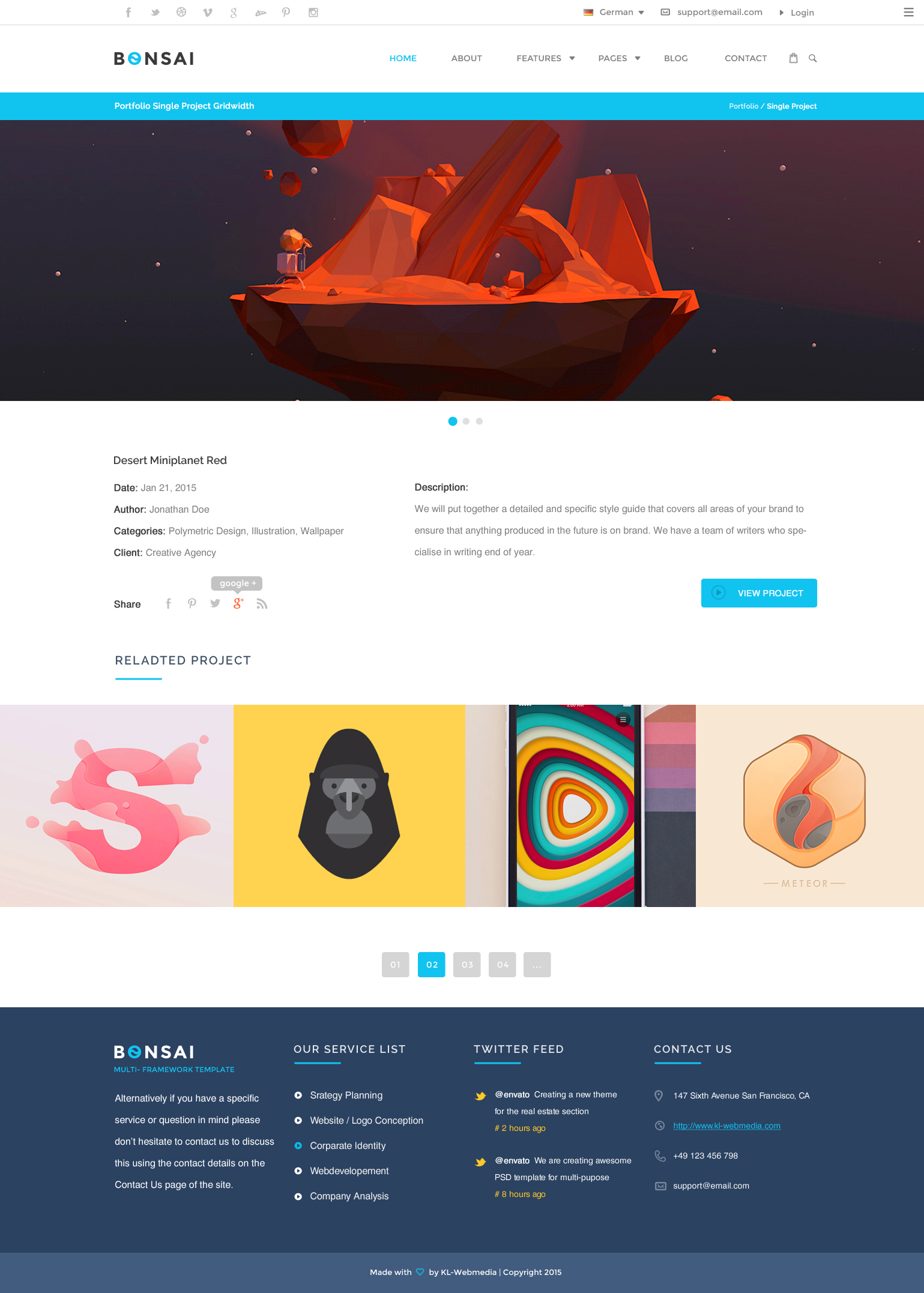**Caption:**

The image features the word "bonsai" prominently displayed at the top left against a white background. Below this, a thick blue line divides the top section from the rest of the background, which showcases a floating island composed of red clay-like rocks. The text "Desert Mini Planet" is inscribed, along with the date "January 21st, 2015," the author "Jonathan Doe," and the categories "Polymatic Design, Illustration, Wallpaper." This project was created for a client named "Creative Agency" and is tagged with the option to share or view related projects.

The image also includes several elements and shapes: an 'S', a swirling monkey, a guitar pick-shaped object with paint shaded colors, a geometrical structure featuring a black planet, and a pink, meat-colored object.

A description within the image states, "We put together a detailed and specific style guide that covers all areas of your brand to ensure that anything produced in the future is on brand. We have a team of writers who specialize in writing end-of-year review projects."

At the bottom, the image reiterates the word "bonsai" along with sections titled "Our Service List," "Twitter Feed," and "Contact Us." It also provides energy planning services with an address, phone number, and email contact details.